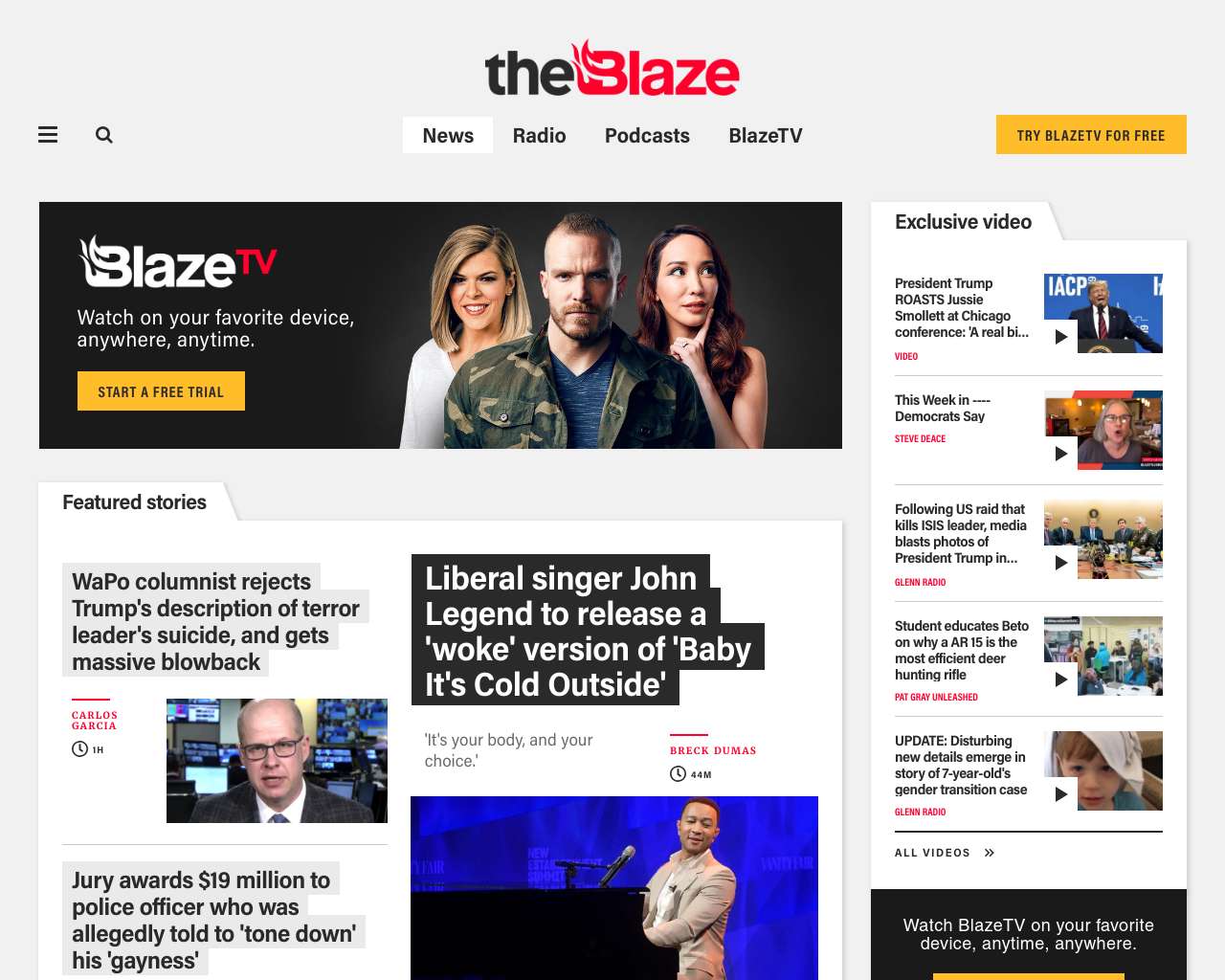Screenshot of The Blaze Website

The screenshot depicts the homepage of The Blaze, a news and entertainment website. The Blaze's logo is prominently displayed at the top of the page, featuring the name "The Blaze" with "The" in black and "Blaze" in red. The 'B' in "Blaze" is stylized to resemble a flame, emphasizing the fiery brand identity.

Beneath the logo are four main navigation tabs: News, Radio, Podcasts, and Blaze TV, each directing users to different sections of the site. In the upper right-hand corner, a bright yellow square prompts visitors to "Try Blaze TV for free," a call-to-action for the site's subscription service.

On the right-hand side of the page, there is a column designated for "Exclusive Videos," showcasing five video thumbnails. Each thumbnail features a play button overlay and a description of the video's content displayed to its left.

Dominating the main content area is a featured story about liberal singer John Legend. The story highlights his release of a modern, "woke" version of the classic song "Baby It's Cold Outside." The article is accompanied by a prominent image of John Legend, categorizing it under the "Featured Stories" section.